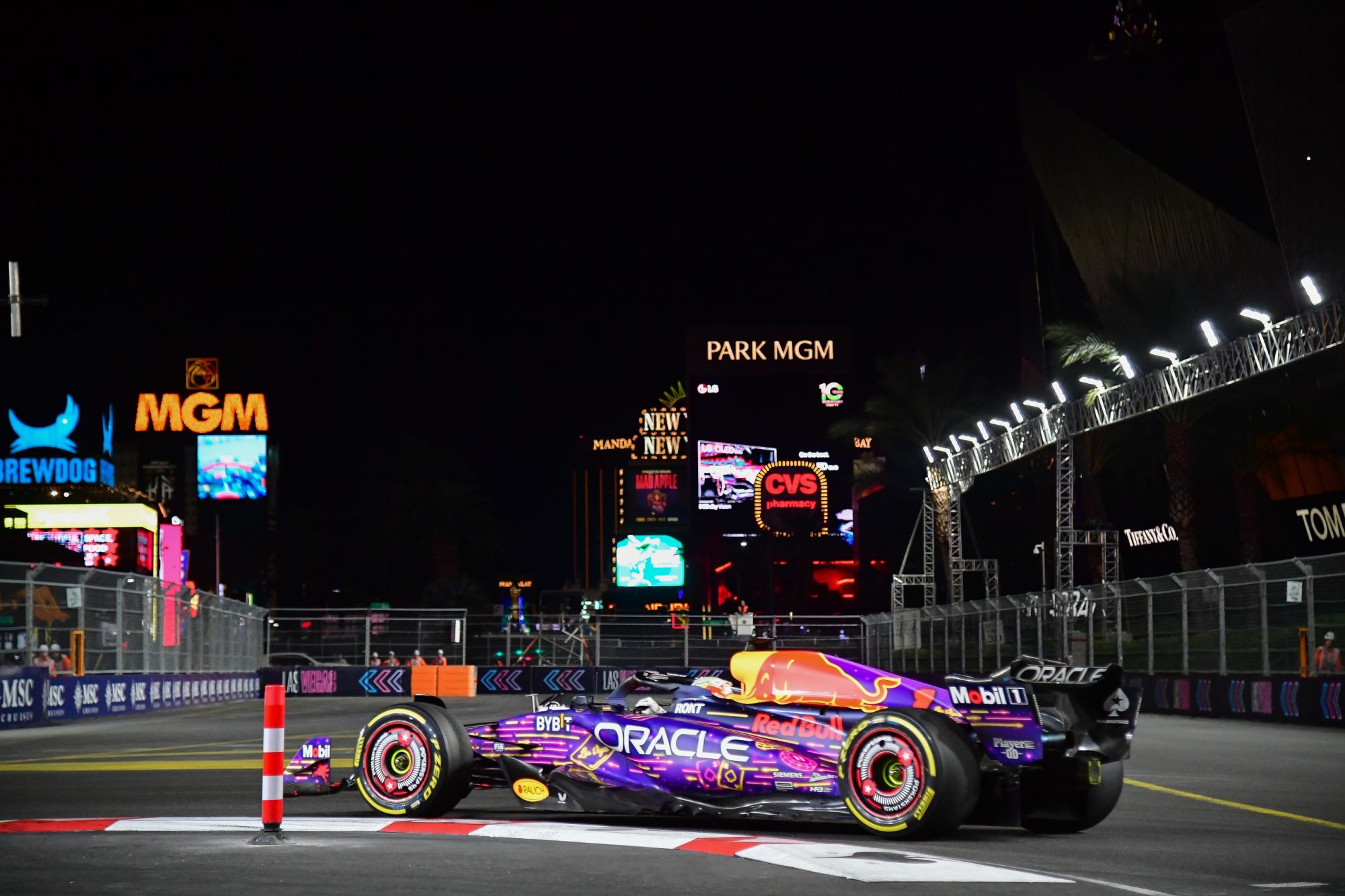This professional nighttime color photograph showcases a striking Formula One race car positioned on a racetrack. Illuminated from above, possibly by studio lighting, the car is accentuated against the dark sky and background. The race car predominantly displays a vibrant palette with bright oranges, yellows, purples, and pink stripes, along with red and white accents on the track. Notably, the vehicle features prominent branding, with "Oracle" written on the tail fin and central body, and the iconic Red Bull logo on a yellow background. Surrounding the racetrack, a fence displays various logos including MSC. In the backdrop, the brightly lit buildings exhibit numerous logos such as MGM, Park MGM, BrewDog, CVS Pharmacy, and Tiffany & Co. A red and white line runs along the bottom of the track, converging towards the vehicle, and additional signage and lights create a vivid contrast against the night sky, further enhancing the scene’s dynamic and detailed visual composition.